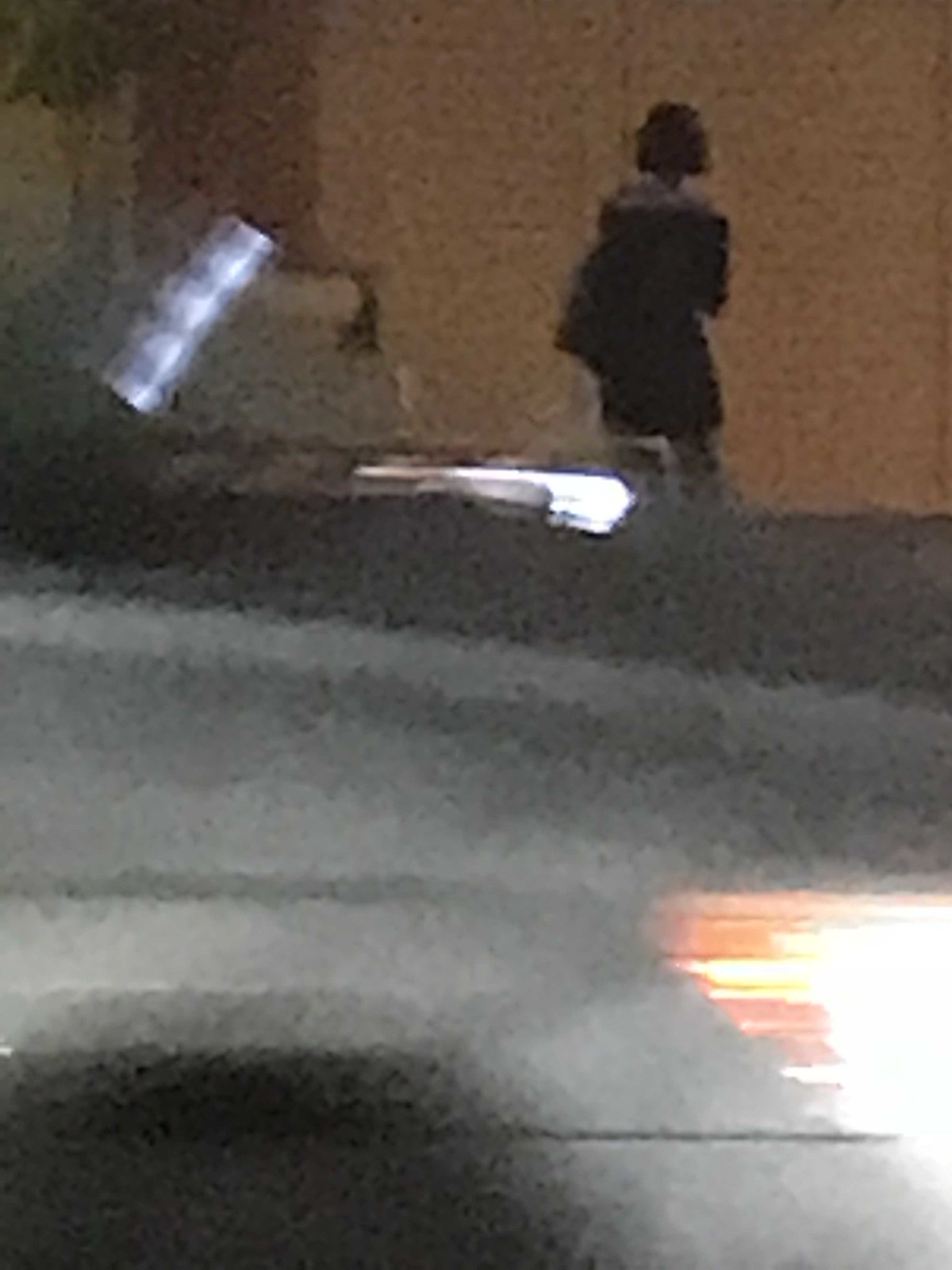A grainy, out-of-focus nighttime photograph captures what appears to be a zoomed-in image of the front side of a grey metal car. The visible portion includes the bonnet, wheel arch, and a black semi-circular tyre. The headlight is prominently bright white at the front with an orange light trailing behind it. In the background, a light-colored wall is visible along with a woman standing, facing away from the car. She has short, possibly curly, black hair and is dressed in a black coat that may have a hood or scarf. She appears to be carrying a bag and wearing trousers. To the left of the frame, there's a reflective light or a long cylindrical object diagonally bisecting the image, which is challenging to clearly identify due to the graininess and poor focus.